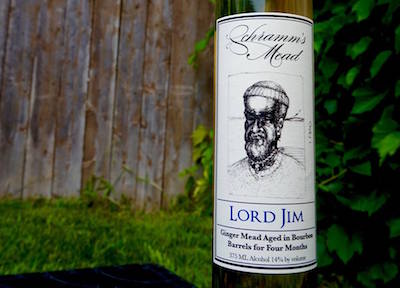The image features a cylindrical glass bottle of Schumann's Mead, positioned outdoors against a backdrop of green grass, a wooden fence, and some trees. The bottle has a greenish tint and a prominent white label. At the top of the label, "Schumann's Mead" is elegantly written in cursive black lettering. Centered on the label, there is a hand-drawn, black-and-white sketch of a bald-headed man with a headdress, portraying a character named Lord Jim. His image has a pencil sketch quality, adding a vintage feel. Below the drawing, the name "Lord Jim" is inscribed in blue text. Further down, the label specifies "Ginger Mead aged in bourbon barrels for four months" in black text. Additionally, the label includes details on alcohol content and volume, although the specifics are not clear. The scene behind the bottle features lush greenery, including bushes and a wooden fence composed of weathered, thin slats that have turned a grayish color over time.